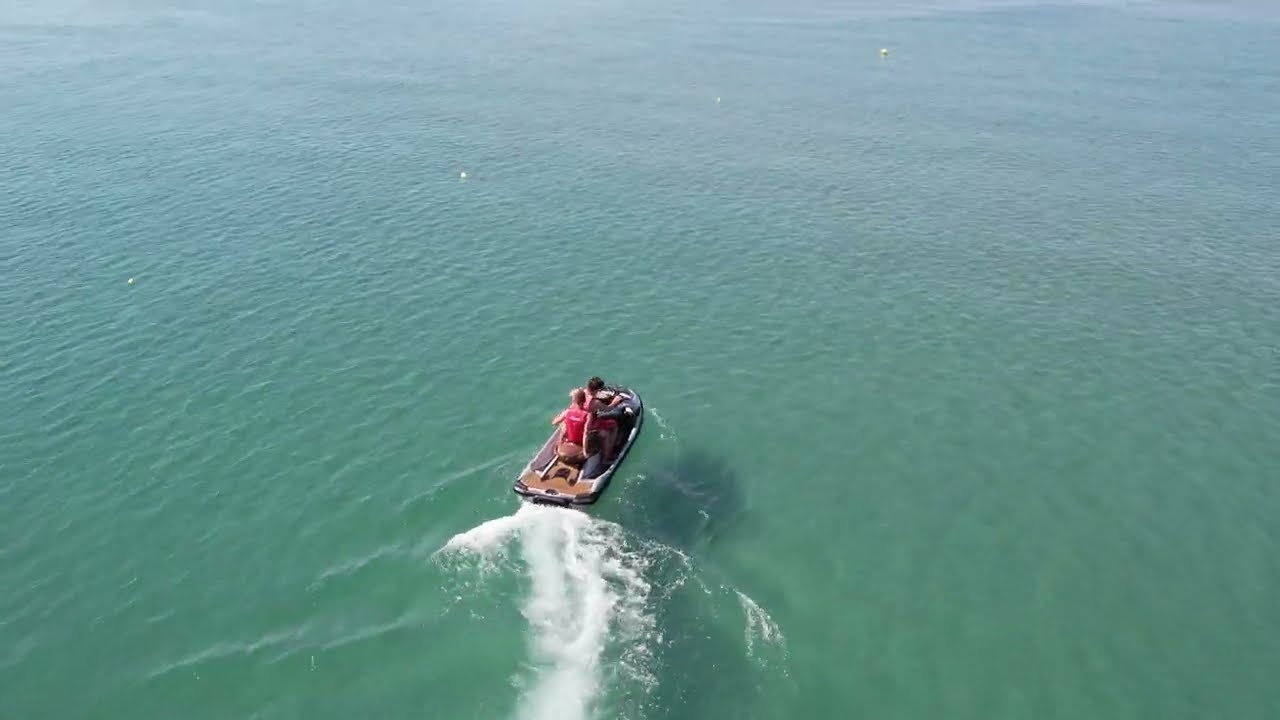A vibrant photograph taken on a partly cloudy day captures the excitement of two people on a small, white and brown speedboat, cutting through a clear, turquoise ocean. The boat, positioned toward the bottom center of the image, leaves a foamy white trail in its wake. The duo, likely a male driver and a female passenger, are both clad in red, possibly life jackets, and are heading toward the upper part of the image, back facing the camera. The sun is almost directly overhead, casting a distinct shadow of the boat onto the ocean floor, which appears shallow and semi-transparent. The water is a mesmerizing mix of blue and green hues, revealing its clarity. To the upper left of the scene, a line of four white buoys floats on the surface, acting as markers, indicating the path the boat is approaching. The image combines the dynamic movement of the boat with the serene backdrop of the vast ocean and the softly lit sky.